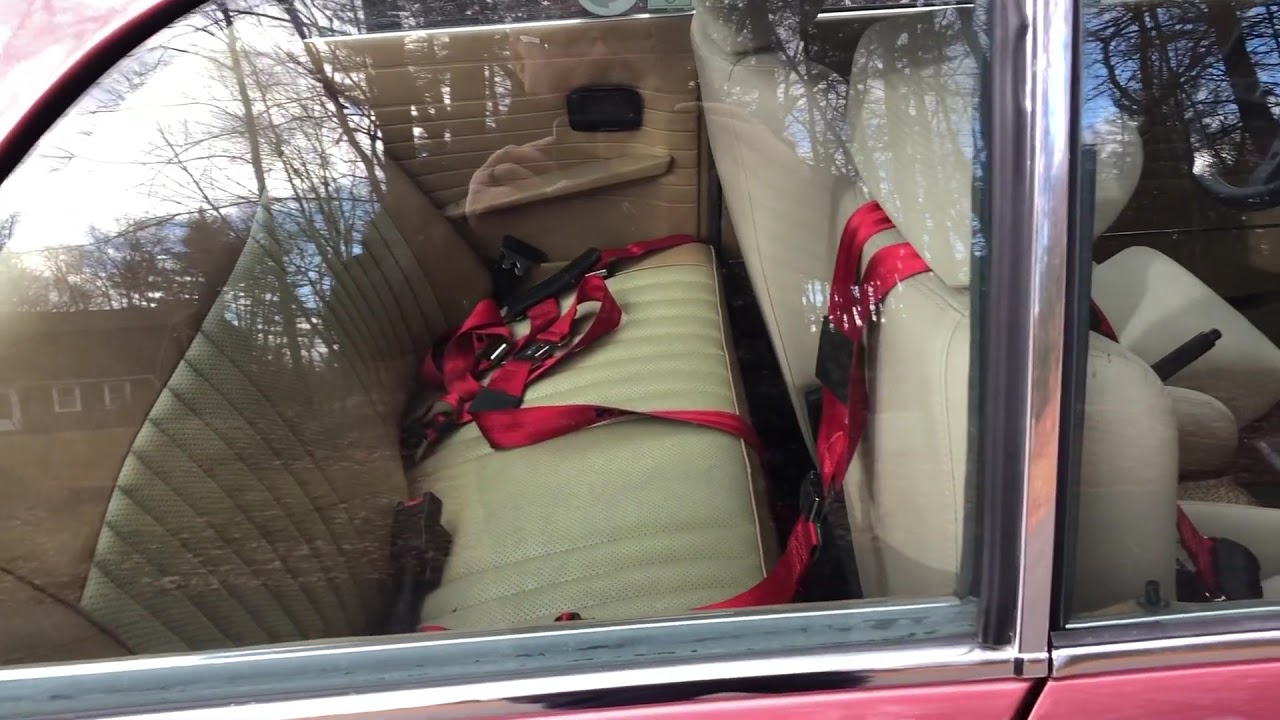The photograph, taken from outside a vehicle through its windows, features a horizontally aligned rectangular view showcasing a cream-colored interior. The focus is on the back seat, a beige or ivory-colored bench-style seat made of leather or vinyl, with several red and black lap belts lying across it. The left side of the image emphasizes the back seat and the matching door panel, while the right side gives a glimpse of the front seat and part of the front passenger side window. The exterior of the car, visible at the bottom right corner, appears to be pink or possibly red, complemented by silver window frames. Reflections of trees and a house are visible on the window surfaces, adding a textured dimension to the scene.